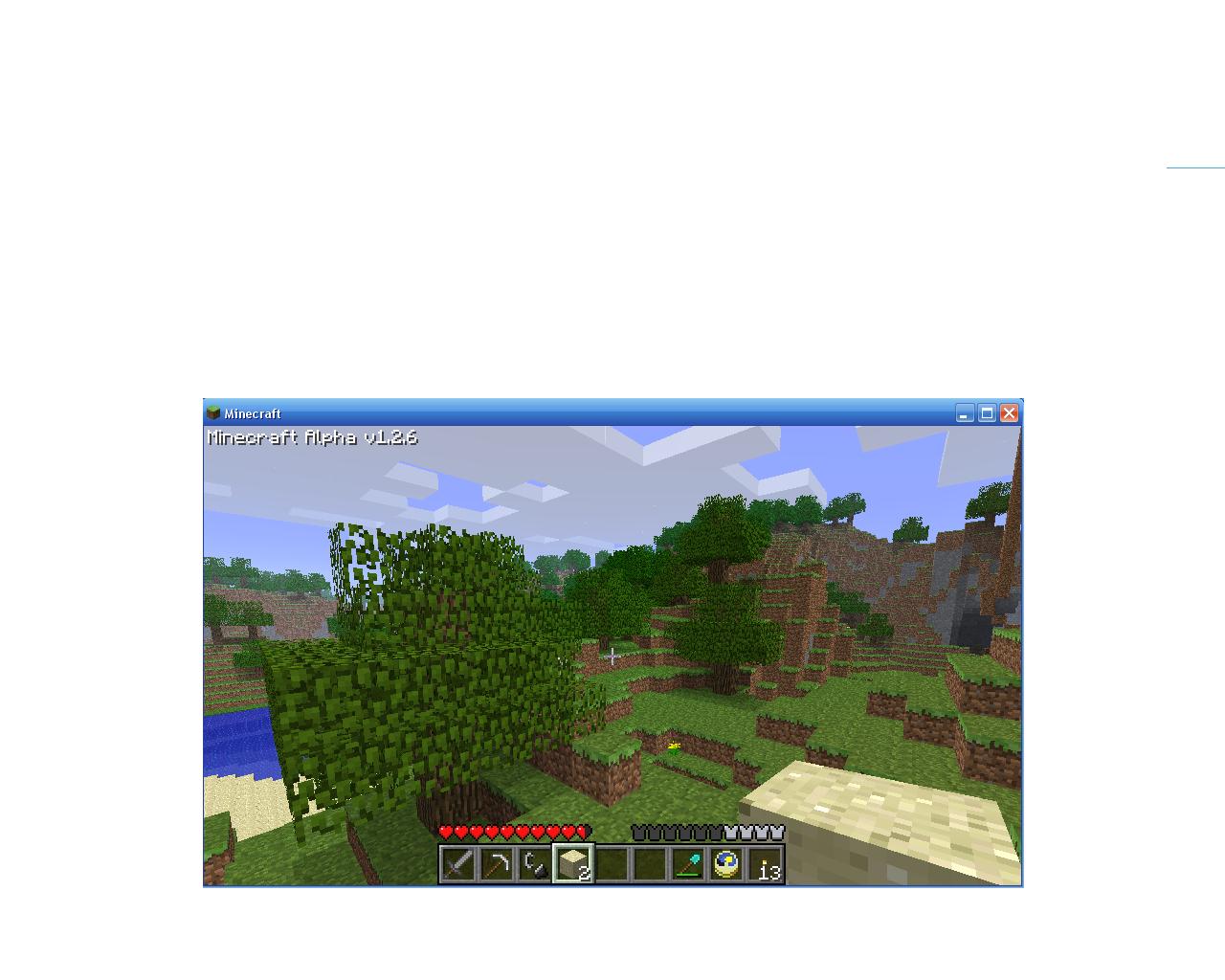The image depicts a screenshot from the video game "Minecraft," specifically from its Alpha version 1.2.6, as indicated by the white text in the upper left corner against a light blue background. The screenshot is captured on a computer screen, evidenced by the presence of the minimize and close buttons in the upper right corner. The in-game scene showcases a landscape composed of multiple green, grassy levels layered upon the earth, characteristic of Minecraft's blocky terrain. In the lower right corner, the player's score is displayed as 13. The bottom of the screen shows the player's health in the form of hearts, with approximately eight or nine visible. Additionally, there are icons resembling the shape of t-shirts, with four light gray and seven dark gray ones, possibly indicating armor status or inventory items.